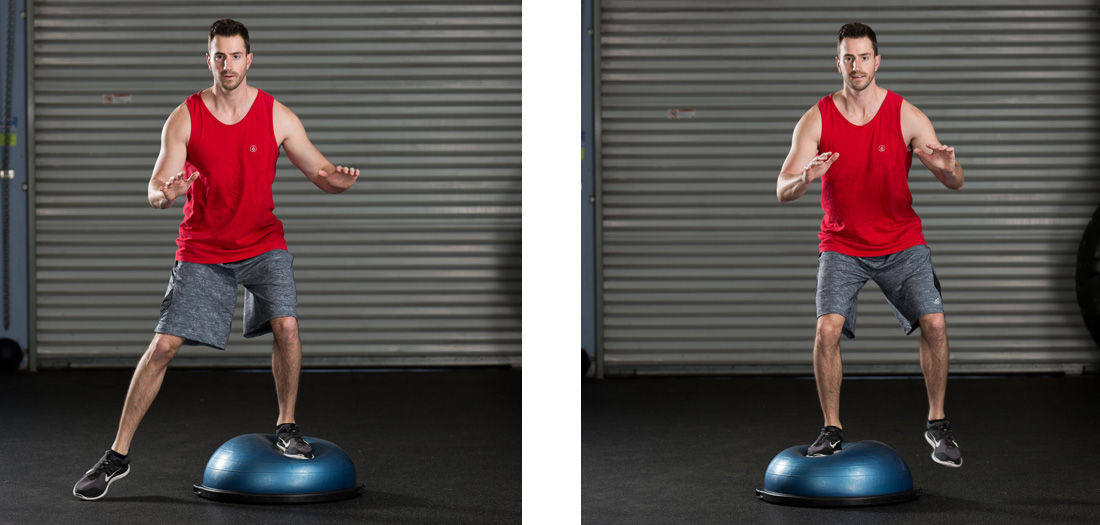The image shows two side-by-side photographs of the same man standing on a black floor, performing balance exercises against the backdrop of a gray, slatted surface resembling a garage door. The man is wearing a red sleeveless tank top, gray shorts, and black and white sneakers. Both images feature a blue half-exercise ball, used as a balance training device.

In the left photograph, the man balances with his left foot on the blue exercise ball, raising his bent arms to shoulder height, palms facing downward, while his right foot remains grounded. In the right photograph, the positions reverse: his right foot rests on the exercise ball with his left foot up in the air, and his bent arms remain lifted. Both images emphasize his active engagement in maintaining stability on the exercise device.